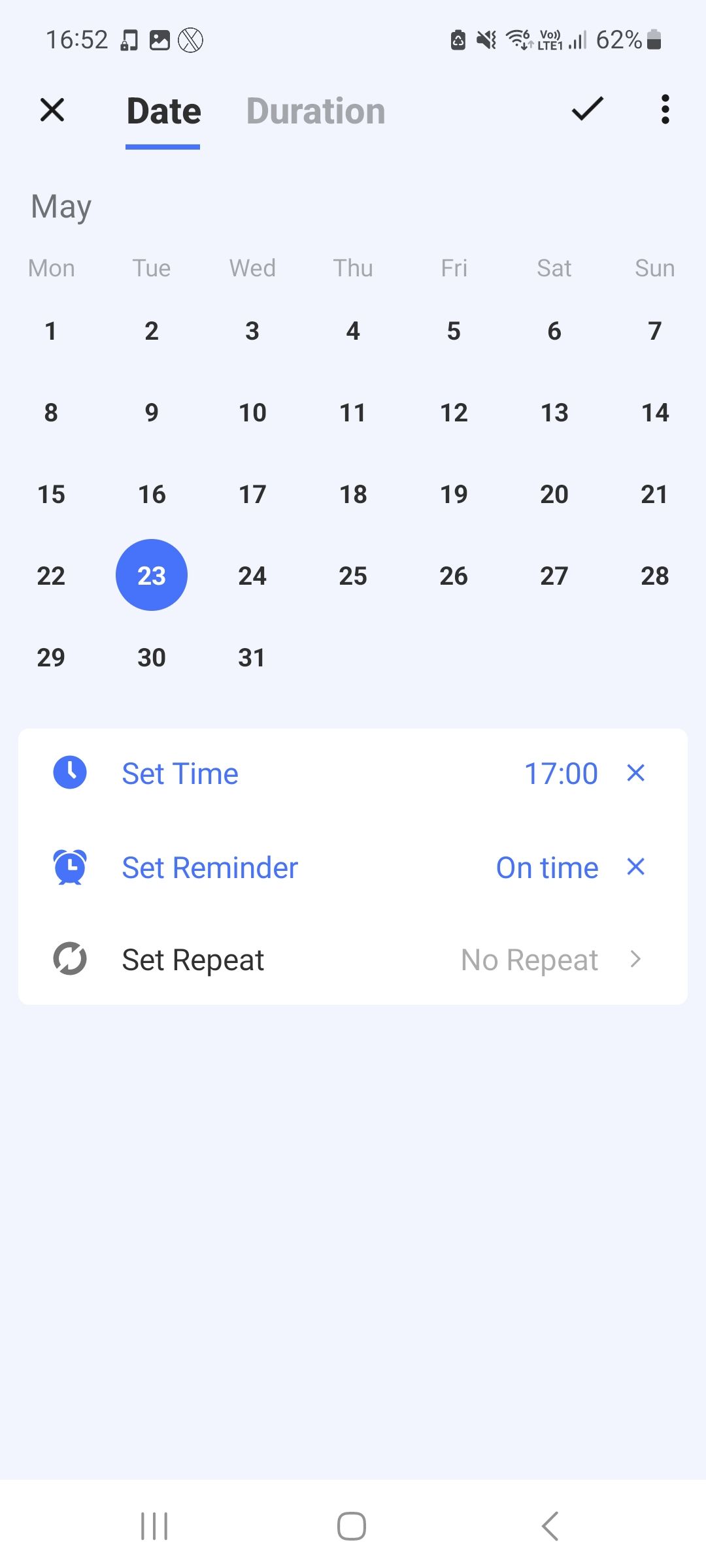This screenshot captures the calendar interface of a smartphone app, depicted against a backdrop of a very light blue, almost white. In the top left corner, there is a black "X" icon. Just to its right is a bolded, black current date, underlined in blue. Further right, there is an indication of the event duration in dark gray text. On the top right corner, there are three vertically aligned black dots.

Below the black "X", the text "May" is displayed in a slightly darker gray. Directly underneath this, the days of the week are listed from left to right: Monday, Tuesday, Wednesday, Thursday, Friday, Saturday, and Sunday. Beneath these labels, the calendar dates are displayed, with Monday as the 1st and Sunday as the 7th, continuing up to the 31st which falls on a Wednesday. All the numbers are in black, except for the 23rd which is highlighted with a blue circle, and the number itself is white.

Below the date display, there are white rectangles housing various icons and options. The first rectangle from the top features a timer icon, an alarm clock icon, and a refresh button on the left side, while to the right, it displays "Set time" in blue text. Adjacent to this, a text reads "17:00" alongside a blue "X".

The second white rectangle down reads "Set reminder" with the text "On time" and a blue "X" on the right side. 

The third rectangle reads "Set repeat" in black text. To its right, the text "No repeat" followed by a greater than sign (" > ").

There is a considerable blank space (around three inches) below these options. Centered at the bottom is a gray outlined circle, flanked by three vertical lines to the left and a greater than sign pointing to the right.